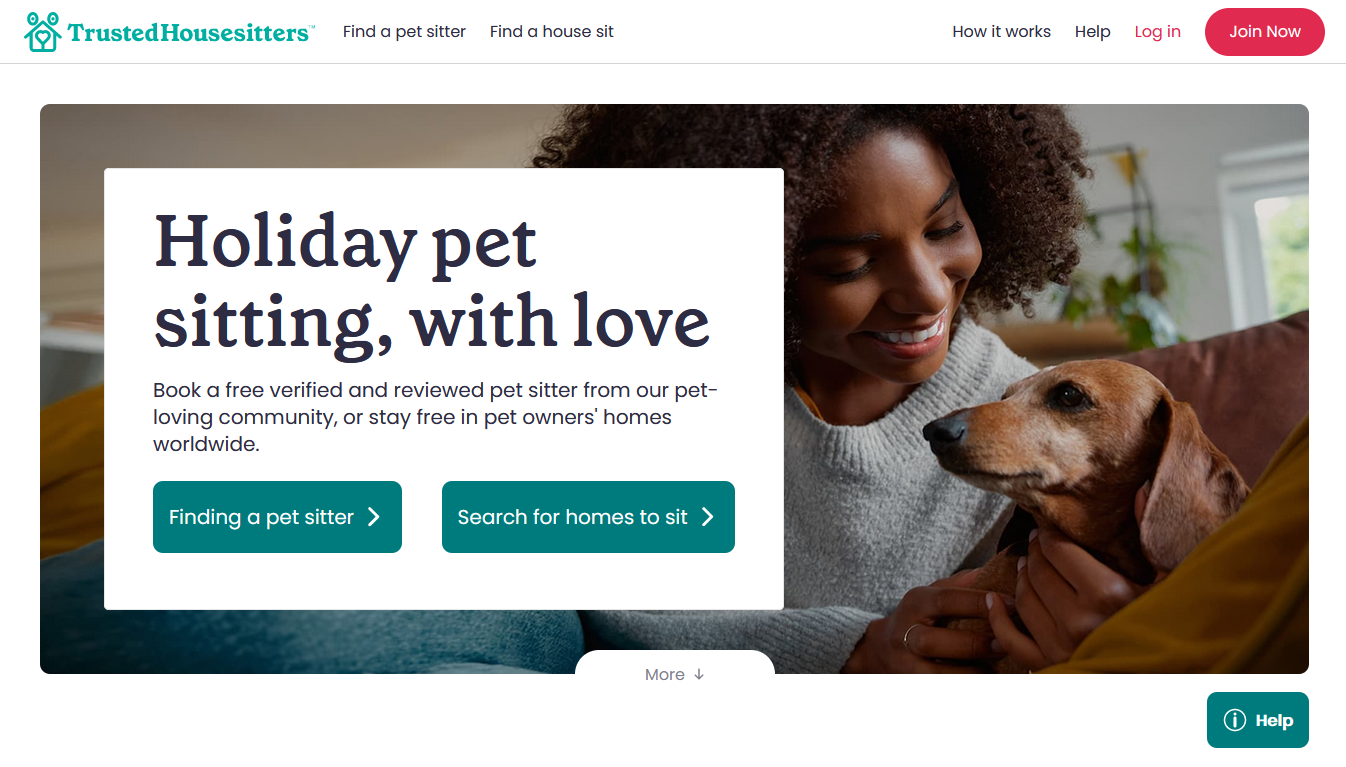The screenshot captures the homepage of the Trusted Homesitters website displayed on a computer. The website has a clean, white background. Central to the page is an inviting image of a woman in a cozy sweater, comfortably seated on a sofa while lovingly holding her dog. Above the image, the banner bar displays the site`s name "Trusted Homesitters" prominently. The banner also offers various navigation options including "Find a Pet Sitter," "Find a House Sit," and additional links for "How it Works," "Help," "Log in," and a prominent "Join Now" button in white text on a red background. 

Overlaying the picture is a white text box that reads, "Holiday Pet Sitting with Love," followed by a brief blurb: "Book a free, verified, and reviewed pet sitter from our pet-loving community, or stay free in a pet owner's home worldwide." Below this informative section, there are two distinct call-to-action buttons. The first, in blue with white text, reads "Find a Pet Sitter," and the second, in the same color scheme, reads "Search for Homes to Sit." This detailed and thoughtfully laid-out homepage clearly guides users towards their desired service, emphasizing trust and community.